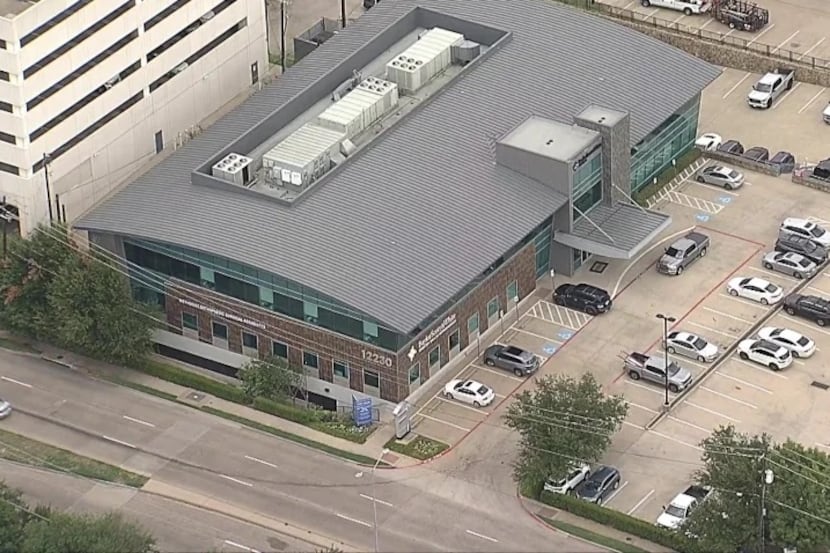The photograph captures an outdoor scene during daytime, viewed from an altitude of approximately one to two hundred feet and oriented horizontally, providing a slightly angled perspective from above. Central to the image is a large, two-story building with a gray, arched roof, which features some glass sides and windows. The building, possibly a medical facility or office, bears the address "12230" prominently in white font. Surrounding the building is a parking lot, situated to the right, which is roughly half full with various cars and trucks. This parking area is bordered by green trees and set on gray cement with white parking lines. Adjacent to the building, there is a place for easy drop-offs, suggesting accessibility for wheelchair users or handicapped individuals. In the top left corner of the image, a taller white structure, likely a parking garage, is visible. The bottom portion of the photograph includes a street running left to right, alongside which there is a sidewalk flanked by more trees and grass, adding to the verdant surroundings. Utility or industrial equipment can be seen on the building's roof, possibly serving as energy or generator units.